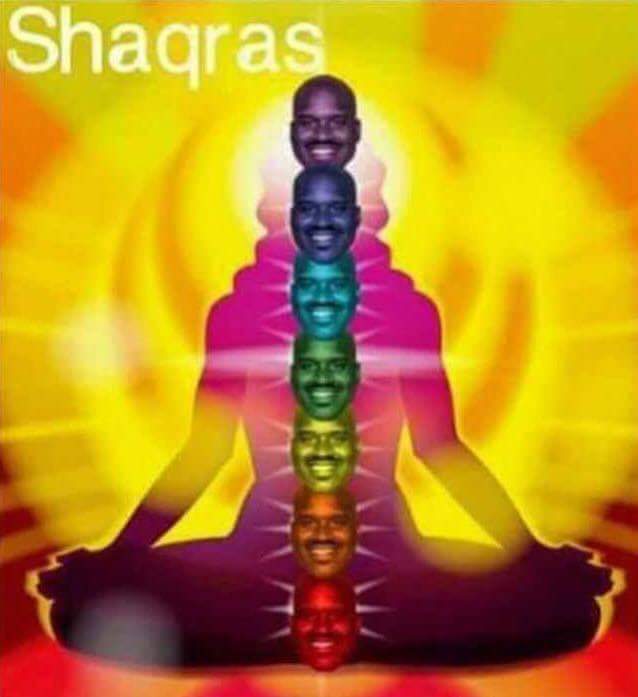This whimsical image features a person sitting in a classic Lotus pose, meditatively crossing their legs with hands resting on their knees. The background showcases a vivid, creative sunburst pattern dominated by yellow and orange hues. Superimposed over the meditative figure is a vertical stack of seven smiling faces of Shaquille O'Neal, rendered in a totem-like style. Each face is a different color, creating a rainbow effect: starting with red at the bottom, followed by orange, yellow, green, light blue, dark blue, and purple. To add to the playful tone, the top left corner features white text spelling "Chakras," cleverly blending Shaquille O'Neal's name (spelled "Shaq," S-H-A-Q) with the spiritual concept of chakras. This image humorously juxtaposes the serene practice of meditation with a light-hearted, colorful twist.